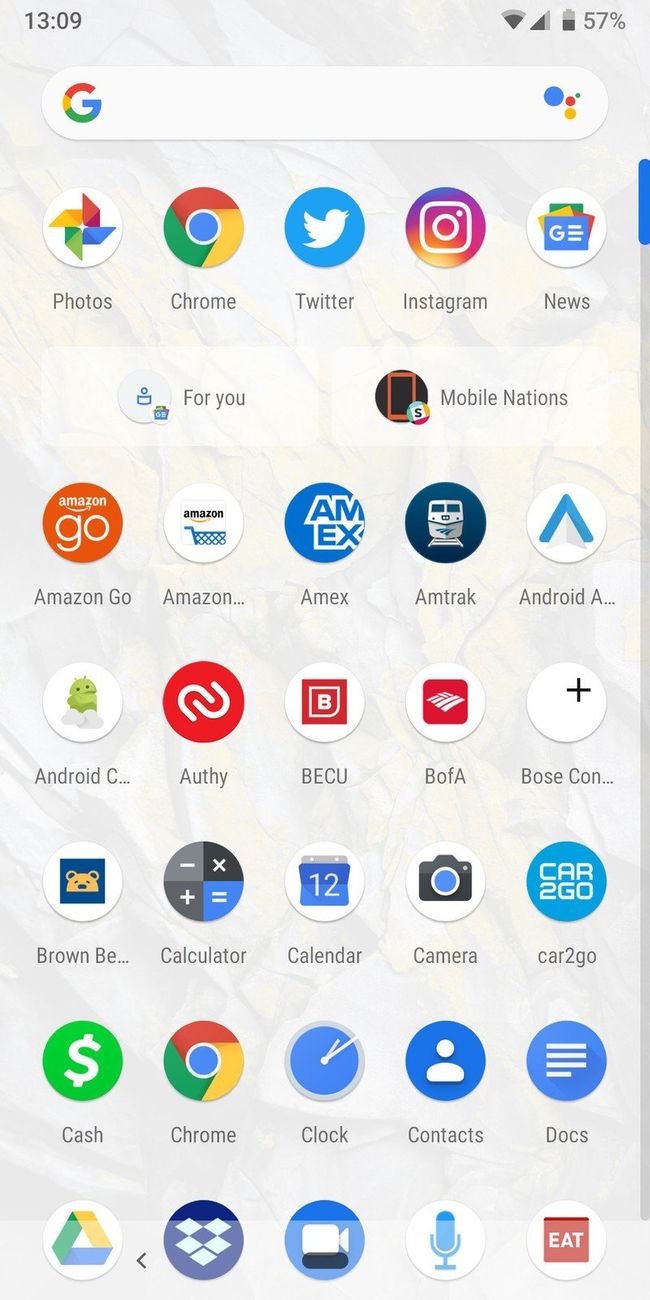The image showcases a screenshot of a smartphone's home screen, which appears to be that of a Google Pixel phone. The screen has a predominantly white and gray background adorned with a multitude of vibrant app icons, typical of Google's color scheme that includes hues of red, blue, green, and yellow. 

At the top of the screen, the familiar multicolored 'Google' logo is clearly visible. Below it, a variety of app icons are neatly arranged and span across several rows. Some of the notable icons include:
- Photos
- Chrome
- Twitter
- Instagram
- Google News
- For You
- Mobile Nations
- Amazon Go
- Amazon
- MX
- Amtrak
- Android
- Bank of America
- BECU
- Calculator
- Calendar
- Camera
- Car2Go
- Cash
- Chrome
- Clock
- Contacts
- Docs
- Microphone
- Uber Eats
- Film

Each icon is distinct, contributing to the overall colorful and user-friendly interface.

The time displayed is in military format, reading 13:09 (1:09 PM). The battery indicator shows a 57% charge remaining. There are approximately 30 to 35 different icons spread across the smartphone’s home screen, presenting a comprehensive and organized layout typical for an Android device.